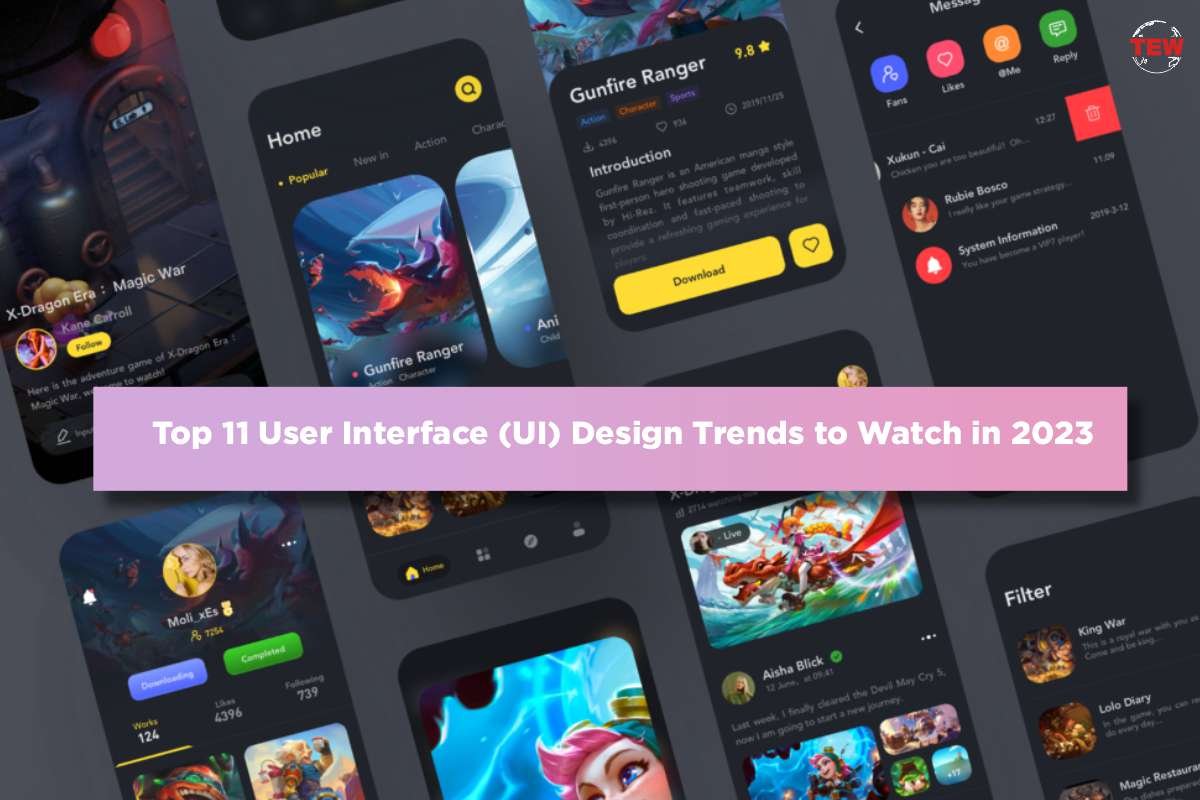The image displays a promotional ad or a YouTube video thumbnail featuring a central purple-pink gradient box with white text that reads, "Top 11 User Interface (UI) Design Trends to Watch in 2023." Surrounding this central banner are nine different screenshots of mobile user interfaces, giving a collage-like effect. 

The top left screenshot showcases an app called "X-Dragon Era: Magic Wars," suggesting a fantasy game interface. Below it, another interface belongs to a user named "Molly_XES," who has 124 works. Another prominent screenshot towards the top center advertises "Gunfire Rangers," including its homepage view and a detailed close-up showing it has a rating of 9.8 stars, along with an option to download or save the game. 

At the very bottom, there is an interface featuring an avatar with pink hair and a blue hat, set against a blue background. Additional screenshots include names and elements such as "Ayesha Black," "Zucon," and a filtering option with categories like King, War, Lolo, Diary, and Magic Restaurant. Collectively, these images illustrate various UI design trends and elements from multiple mobile applications, emphasizing popular and visually engaging interfaces for 2023.